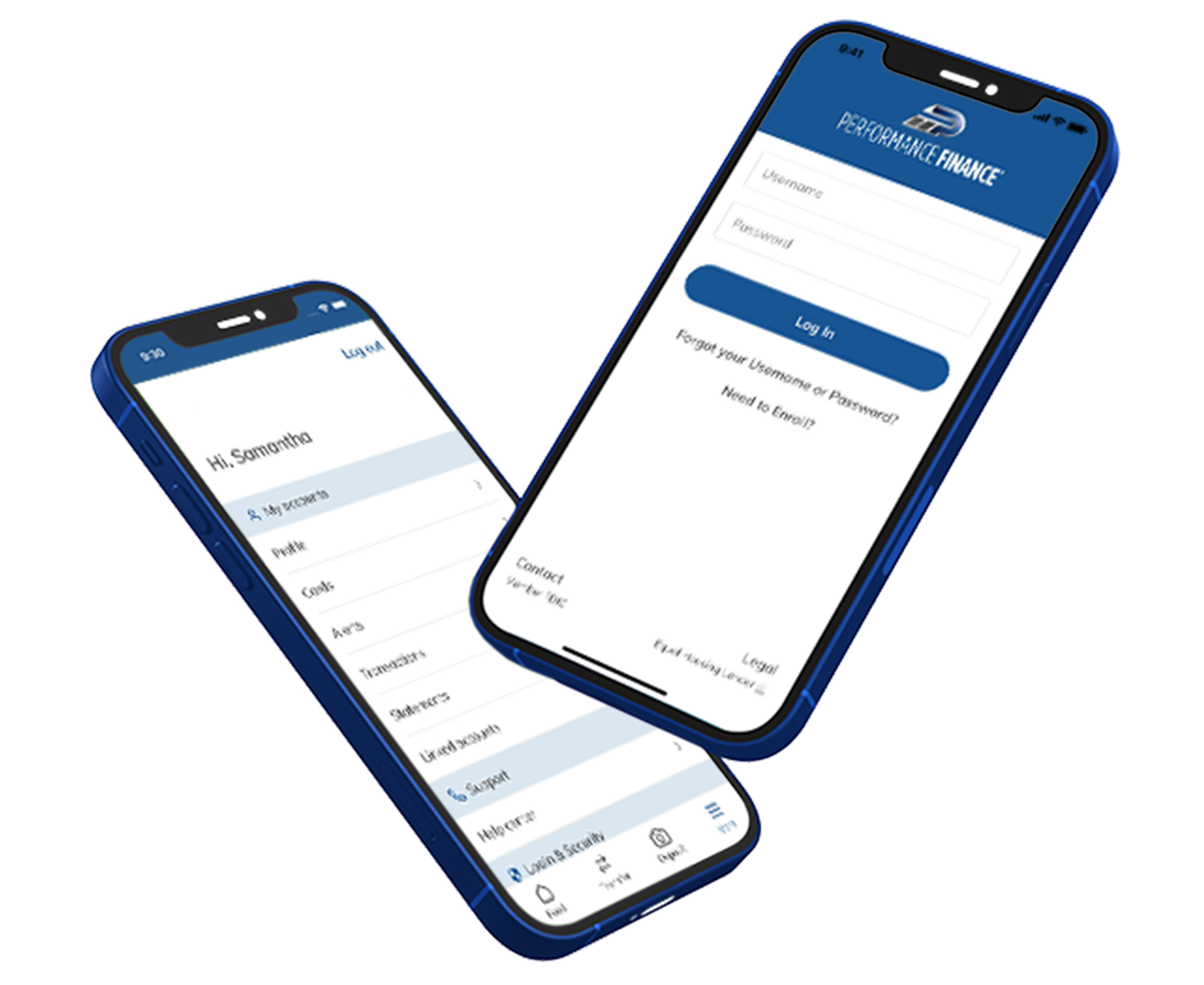This image is a product advertisement showcasing two smartphones seemingly suspended mid-air, artistically angled to suggest motion. Both phones display screens for a financial management app named "Performance Finance," with a distinctive dark blue header. The first phone screen shows the login interface, featuring fields for 'Username' and 'Password,' a blue 'Login' button, and links for 'Forgot your username or password?' and 'Need to Enroll.' The second phone screen reveals the account homepage, greeting the user with "Hi Samantha" and displaying options such as 'My Accounts,' 'Profile,' 'Transactions,' among other partially legible menu items, suggesting post-login functionality. The image effectively emphasizes the app's user-friendly interface and comprehensive financial management features.